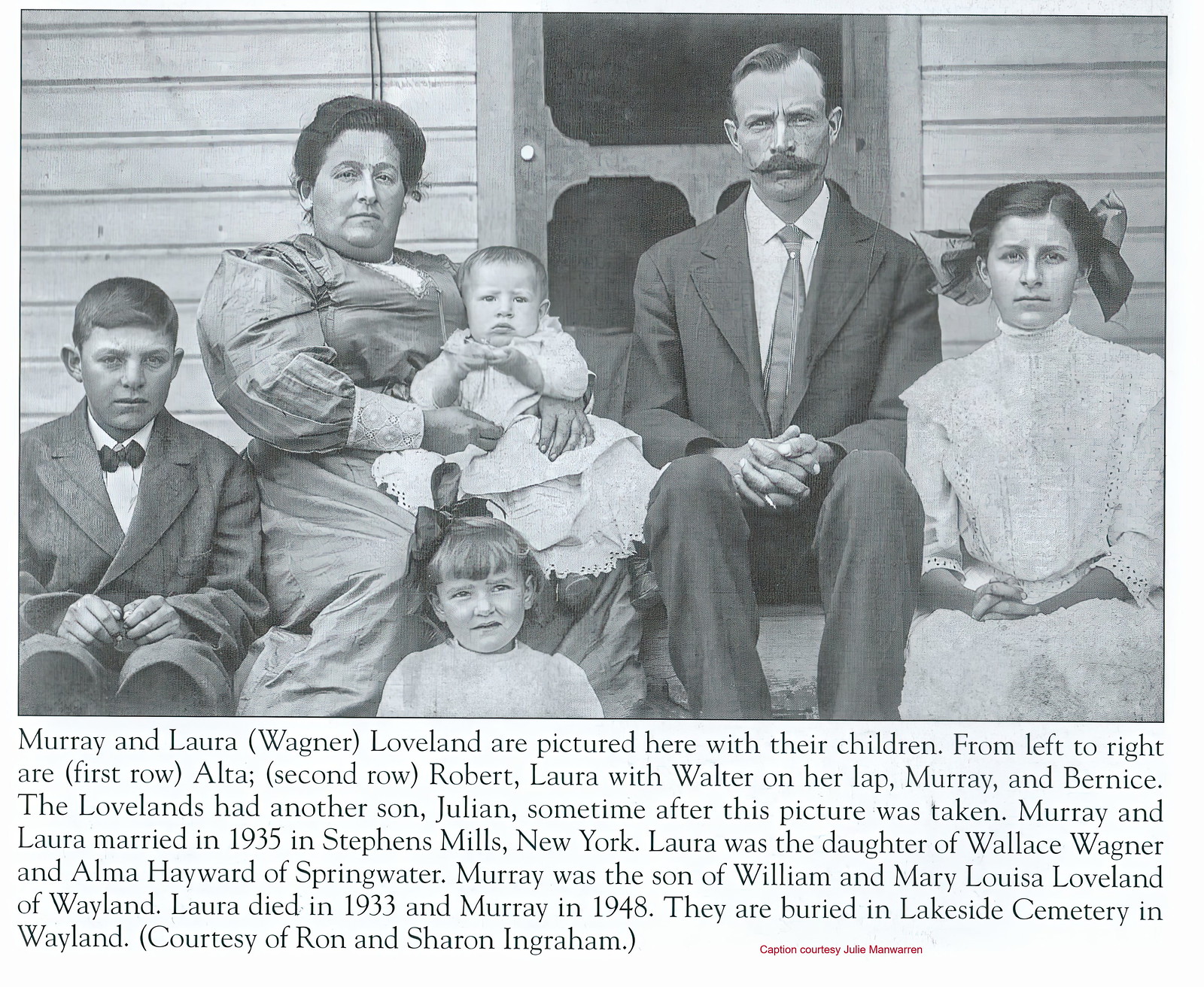This is a black-and-white photograph of the Loveland family, likely from around the early 20th century, based on their attire. The family is sitting on the wooden front porch of their home, which features intricate wood siding and a screen door with rounded windows set into it. The photo contains the parents, Murray and Laura Wagner Loveland, along with their four children arranged from left to right. Alta, the eldest daughter, is approximately 16-17 years old, wearing a white dress, and stands to the right of her father. Murray, the father, sports a long mustache, a black suit, and has his hair parted to the side. On his left is his wife Laura, dressed in a long, poofy dress and holding their infant son Walter on her lap. Laura’s hair is styled in a bun. Seated next to Laura is their son Robert, who is about 10-12 years old, dressed in a suit and bow tie with his hair slicked to the right. In front of Laura, leaning against her legs, is their youngest daughter Bernice, around 4-5 years old, wearing a white dress and a bow in her hair. All members of the family are looking towards the camera. The caption below the photograph reads: "Murray and Laura Wagner Loveland are pictured here with their children. From left to right, our first row, Alta, second row, Robert, Laura with Walter on her lap, Murray, and Bernice. The Lovelands had another son, Julian, sometime after this picture was taken. Murray and Laura married in 1935 in Stephen Mills, New York. Laura was the daughter of Wallace Wagner and Alma Hayward of Springwater. Murray was the son of William and Mary Louise Loveland of Weyland. Laura died in 1933 and Murray in 1948. They are buried in Lakeside Cemetery in Weyland, courtesy of Ron and Sharon Ingram. Captioned courtesy Julie Marwin."